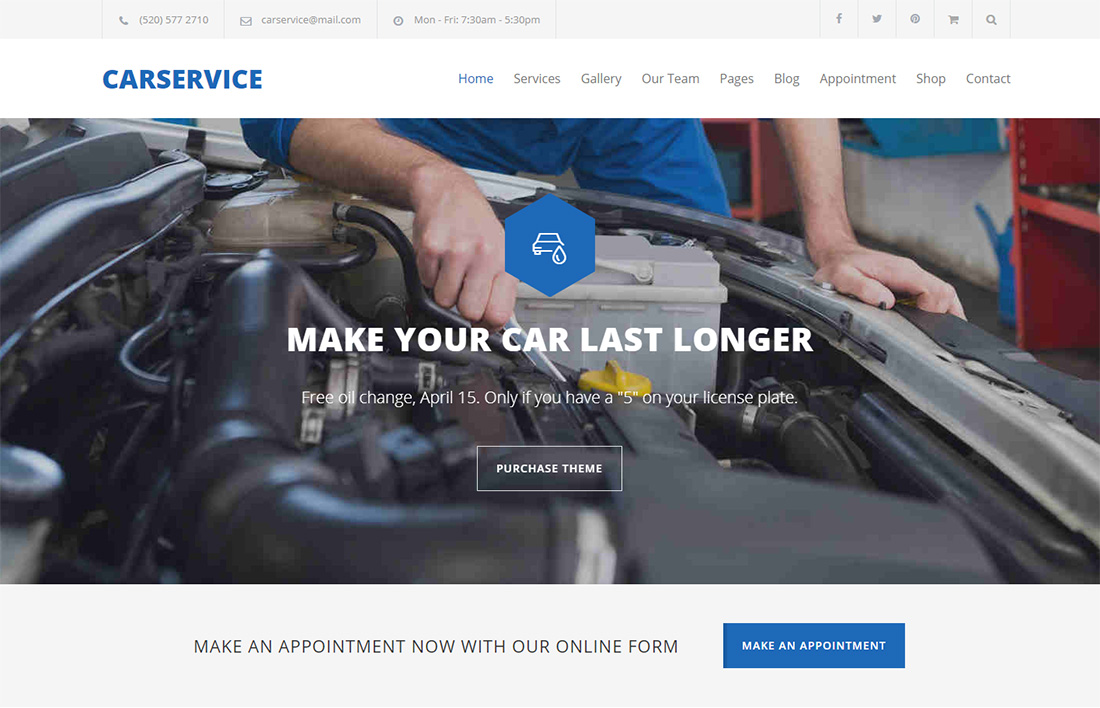The webpage of the car service company is meticulously laid out with essential contact details and navigational elements. At the top left corner, the header displays their phone number, 520-577-2710, followed by their email address, carserviceatmail.com. The opening hours are listed as Monday through Friday, from 7:30 a.m. to 5:30 p.m. On the top right, clickable icons for Facebook, Twitter, and Instagram, along with a shopping cart and a search magnifier, provide easy access to social media and website utilities.

The central focus of the page is a prominent image showcasing a mechanic working on a car, overlaid with a bold message: "Make Your Car Last Longer. Free Oil Change on April 15th, if you have a 5 on your license plate." Beneath this, a transparent button with white lettering labeled "Purchase Theme" invites user interaction.

Above the image, a navigation bar offers links to various sections: Home, Services, Gallery, Our Team, Pages, Blog, Appointment, Shop, and Contact. Below the picture and promotional message, a call-to-action emphasizes, "Make an appointment now with our online form." Next to this text, a blue button with white lettering labeled "Make an Appointment" is prominently placed, encouraging users to schedule their car services. The website is designed to facilitate easy navigation and access to information about car maintenance services, including oil changes and other mechanical repairs.